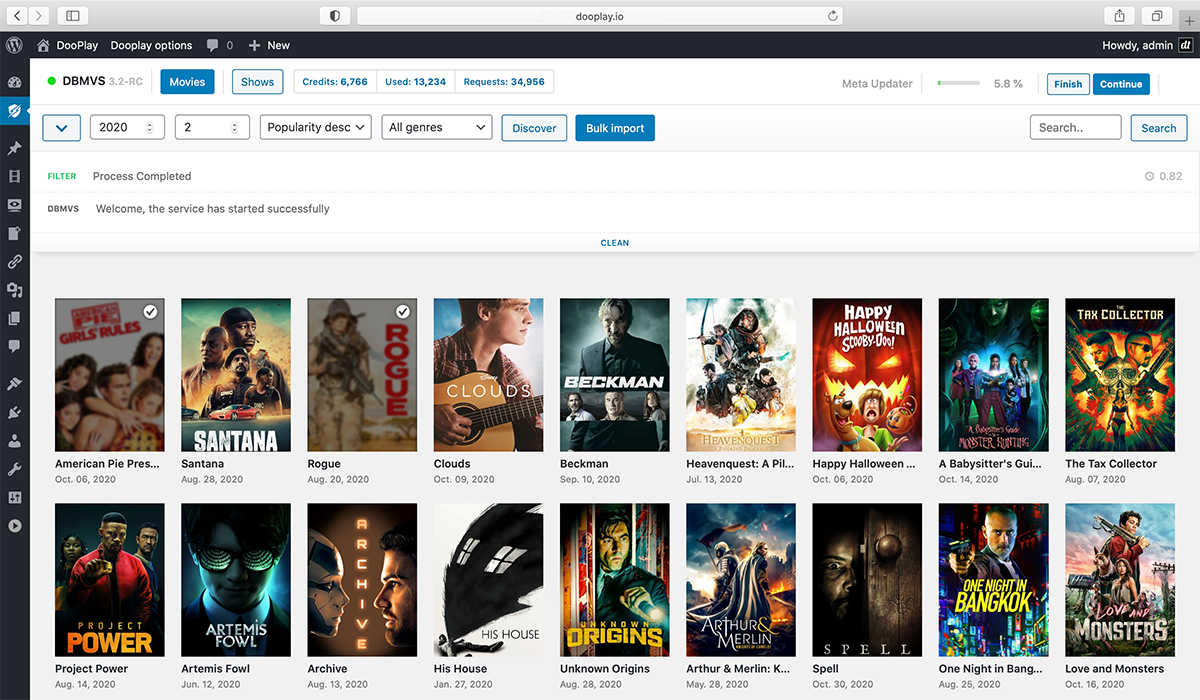In the image, there is a snapshot of the DoPlay website, which features a clean white background. The website display showcases a variety of movie covers prominently. Visible movie titles include "Rogue," "Clouds," "His House," "Archive," "Spell," "Love and Monsters," "Project Power," and "American Pie: Girls' Rules." Each film's cover poster is displayed clearly, making it easy to recognize and select.

At the top of the webpage, there are several filtering options allowing users to search for movies by year, popularity, or genre, aiding in easy navigation. On the left-hand side, small icons represent different functionalities of the website, such as messaging, creating a favorite list, and saving content. There is also an icon that seems to represent user account settings.

The website is branded with the name "DoPlay," which is prominently displayed in the top left-hand corner. The page interface is well-organized, offering an intuitive browsing experience for users searching for films to watch.